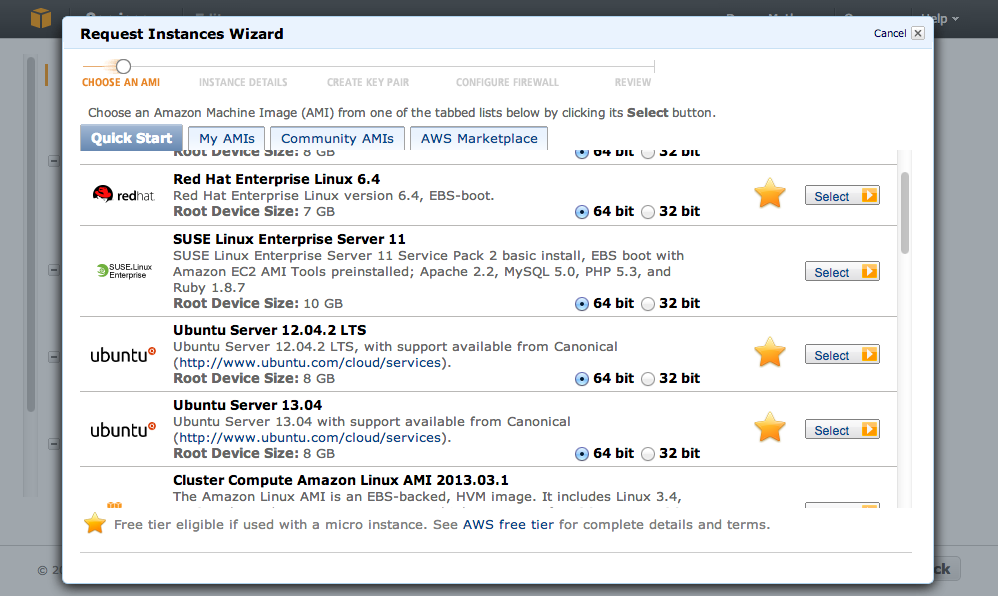The image is a screenshot of a pop-up appearing on a website, where the background page is darkened. The pop-up itself features a light blue header with rounded corners. On the left side of the header, bold black text reads "Request Instances Wizard." To the right, there is blue text labeled "Cancel," followed by a light gray box containing a dark gray "X" icon.

A thin medium blue line separates the header from the main body of the pop-up, which has a white background. In the top left of the main body, a segmented progress bar stretches from near the left edge to about three-quarters of the way to the right. This bar is mostly light gray, except for the initial segment which is highlighted in orange. Positioned on top of the orange section is a white circle with a thin dark gray outline, accompanied by an orange smudge to its left.

Below the progress bar, bold orange text in all caps reads "CHOOSE AN AMI," indicating the current step in the process. To the right of this text, spaced evenly along the bottom of the gray progress line, are the subsequent steps in light gray all caps text: "INSTANCE DETAILS," "CREATE KEY PAIR," "CONFIGURE FIREWALL," and "REVIEW." A thin vertical light gray line marks the right end of the gray progress bar.

Further down, slightly indented gray text provides guidance, stating: "Choose an Amazon Machine Image (AMI) from one of the tabbed lists below by clicking its Select button." The word "Select" is bolded for emphasis, signifying that it is an actionable item.